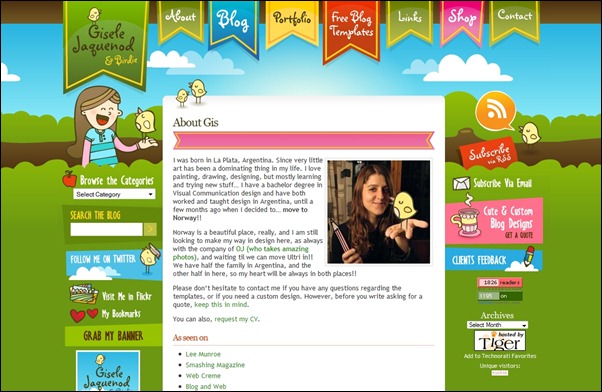The image depicts a vibrant webpage design featuring a variety of colorful elements and details. At the top of the page are tabs shaped like ribbons in various colors, arranged in a horizontal line. The tabs, starting from the top left, include: "Giselle Jaguarnaut and Birdie," "About," "Blog," "Portfolio," "Free Blog Template," "Links," "Shop," and "Contact." The tabs are decorated in blue, green, yellow, red, and pink.

On the left sidebar, the website offers navigational aids and additional features including options to "Browse the Categories," "Select Category," "Search the Blog," "Follow Me on Twitter," "Visit Me on Flickr," "My Bookmarks," and "Grab My Banner." 

The right sidebar includes subscription options such as "Subscribe with RSS" and "Subscribe via Email," alongside promotional sections for "Cute and Custom Blog Design," "Get a Quote," and "Clients Feedback."

The central content of the webpage holds an "About" section, introducing the creator: 
"About Gis: I was born in La Plata, Argentina. From a young age, art has been a dominant passion in my life. I love painting, drawing, designing, and continuously learning new things. I hold a Bachelor's Degree in Visual Communication Design and have both worked and taught design in Argentina. Recently, I moved to Norway, a beautiful place where I am seeking new opportunities in design. Accompanied by OJ, who takes amazing photos, we navigate life with half our family in Argentina and the other half in Norway. My heart is always split between these two places. Please do not hesitate to contact me if you have any questions regarding the template or need a custom design. Before requesting a quote, consider visiting Webcrim, Blog and Web, and Smashing Magazine to view my CV."

The webpage's background is an aesthetically pleasing mix of green, brown, and blue hues, with a sky featuring white clouds, providing a visually appealing setting for the content.